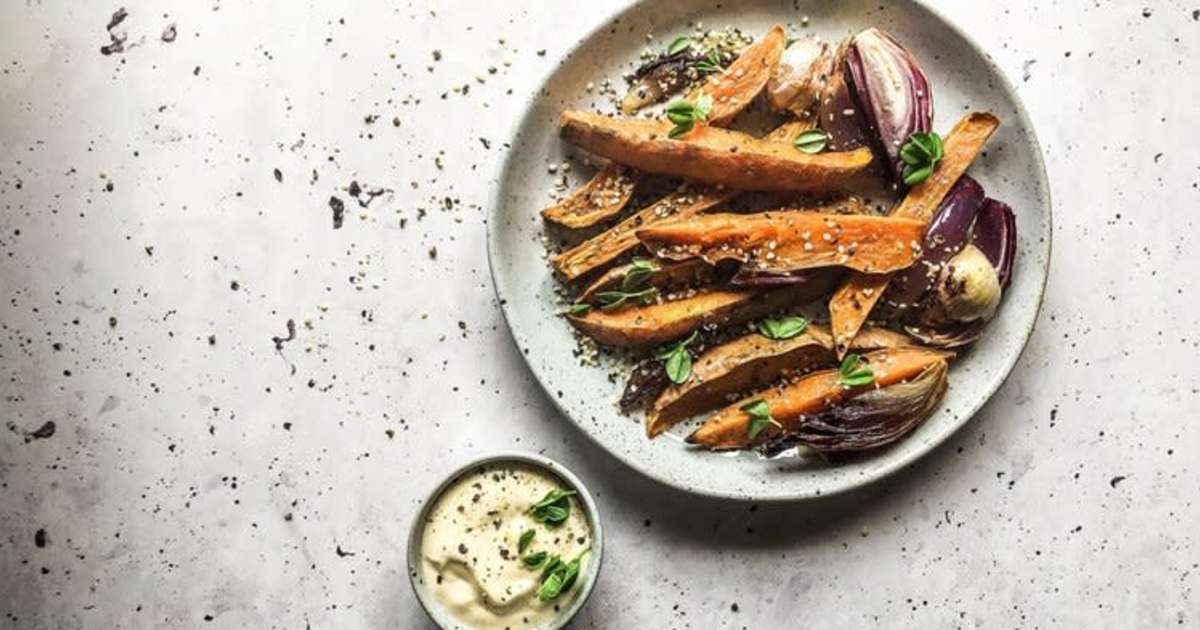This overhead photograph features a fine dining dish centered on a white plate with black speckle marks, mirroring the pattern of the white countertop beneath it. The star of the dish is a serving of natural cut sweet potato fries, with some pieces retaining their skin, imparting a rustic aesthetic. The fries are seasoned and garnished with tiny green herb leaves, likely basil, which add a touch of freshness. Accompanying the fries are chunks of roasted red onion, caramelized to perfection, adding a rich and savory element to the presentation. The dish is complemented by a small ramekin of white sauce, possibly an aioli, also topped with a sprinkling of basil leaves. The entire setting is bathed in natural light, suggesting it was taken next to a window, with a casual scattering of herbs adding to the refined yet rustic appeal of the scene.